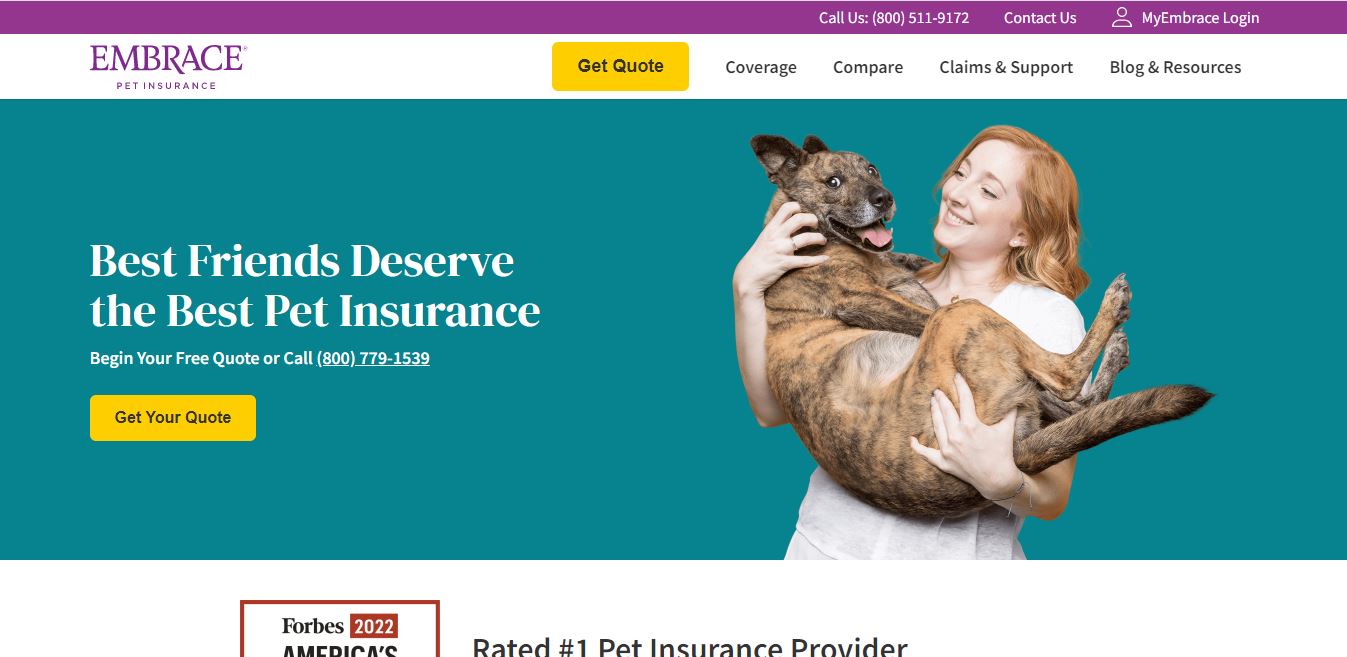A screenshot of a website, taken from a computer screen, capturing the homepage of Embrace Pet Insurance. The top section of the page features a purple bar; the left side is blank, while the right side includes the text "Call Us 800-511-9172" and a "Contact Us" link. In the upper-right corner, there's a "My Embrace Login" option with a small person icon beside it.

Below the purple bar, the main navigation menu includes options such as "Get Quote" in a yellow button next to the word "Embrace," followed by "Coverage," "Compare," "Claims and Support," and "Blogs and Resources." 

Dominating the main section of the webpage is a large blue-green rectangle with a prominent message in white letters stating, "Best friends deserve the best pet insurance." Beneath this, it reads, "Begin your free quote or call 800-799-1539," accompanied by a yellow button labeled "Get Your Quote" in black letters.

To the right of this large blue-green rectangle is an image of a fair-skinned, red-haired woman in white clothing, holding a large brown dog reminiscent of a dingo. The woman cradles the dog in her arms, holding it like a baby with its back resting on her arms and its belly facing up.